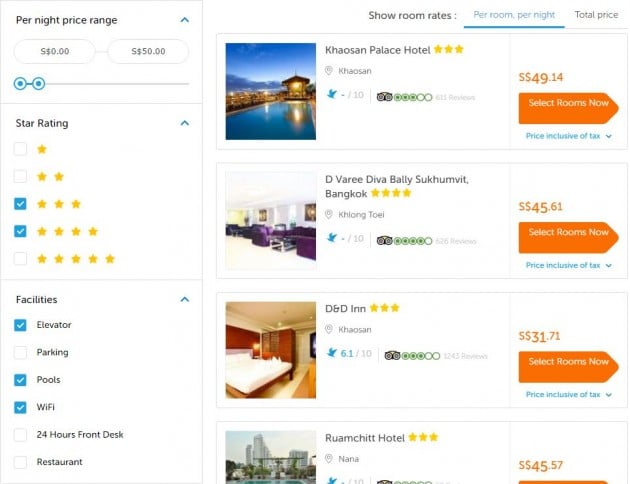The screenshot captures a travel website's hotel search results page, yet the website's branding is not discernible. The sidebar on the left allows users to filter by nightly price, ranging from $0 to $50, and select star ratings, specifically three and four stars, likely due to budget constraints precluding five-star options. The filter options also include desired facilities like elevators, pools, and Wi-Fi, while amenities such as parking, 24-hour desk service, and an on-site restaurant are not prioritized.

Four hotel listings are visible, though the fourth is partially cut off. The first, Kasu-san Palace Hotel, is a three-star hotel priced at $49 per night, featuring a picturesque night scene with the moon and sun reflecting over water. The second listing, Diwari Diva Valley Sakhvalpeta, is a four-star hotel costing $45.61 per night, showcasing a room with purple furniture in its small thumbnail. The third option, D&D Inn, also a three-star hotel, is priced at $31.71 per night and displays a tidy room with a large bed and TV stand. The fourth listing, Ramchit Hotel, three stars at $45 per night, has its thumbnail cut off, rendering the image unviewable.